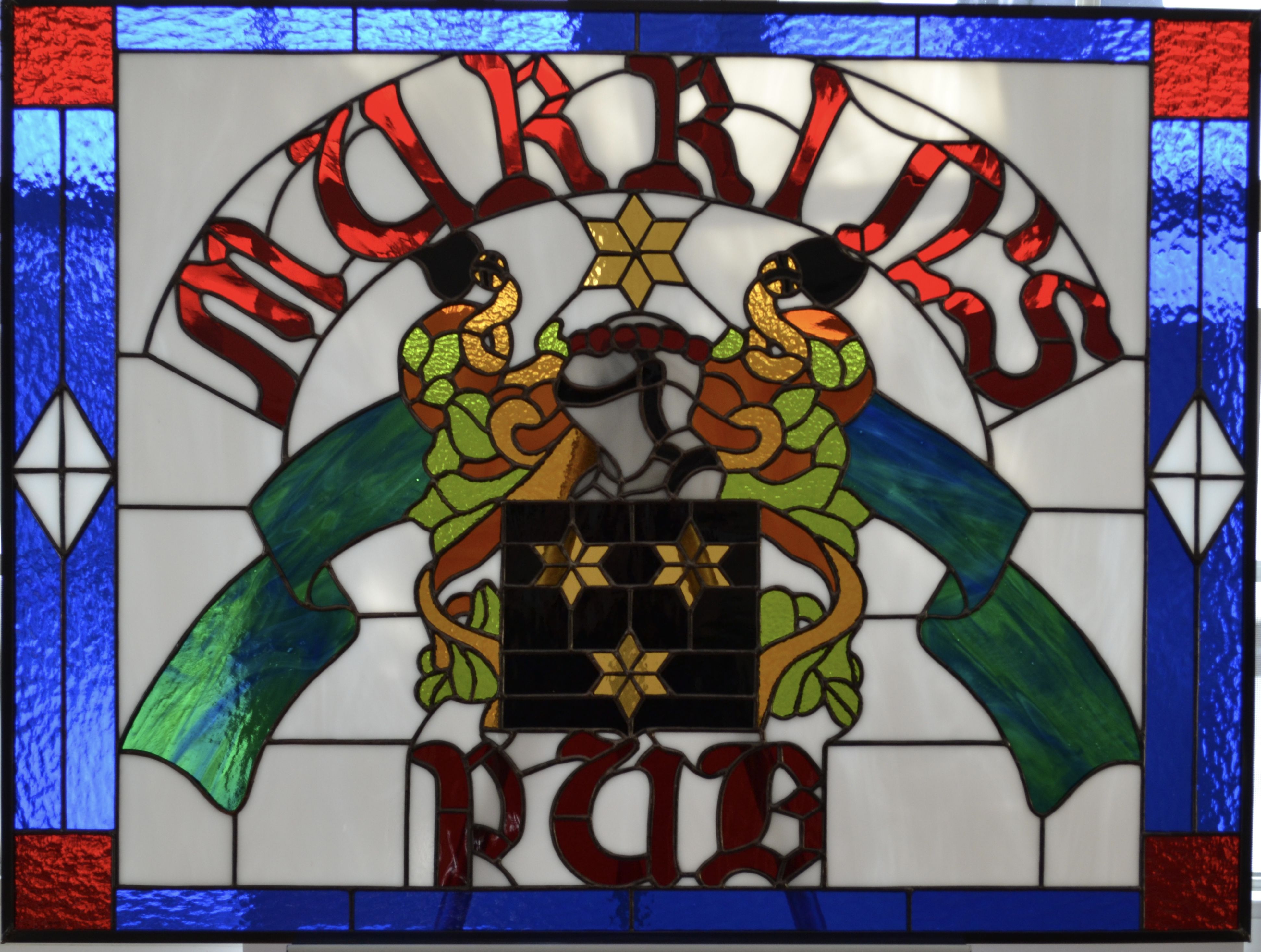This image features a detailed stained glass window from an Irish pub named Merin's Pub. The window is bordered by straight lines of dark blue glass, interspersed with red squares at each corner. The vertical sides of the border have white diamonds with black line crosses that stretch to the top and bottom of the blue sections. In the center of the window, red text with a black outline forms an arch at the top, spelling "Merin's," while the word "Pub" appears at the bottom in matching text. Between the words, there is a black square with three gold stars arranged in a triangular formation. Dominating the central design are two women in brown and olive green, woven into the glass, with a green banner and a knight's head adorned with a red band and additional green detailing. The primary colors throughout the window are blue, red, green, and brown. Light shining through the textured glass provides a sense of privacy by obscuring details beyond the stained-glass artistry.